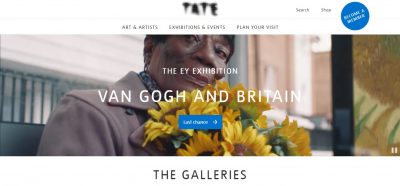Promotional poster for an art exhibit: 

The image features a person seated on a bench, holding a bouquet of vibrant yellow daisies near their chin, giving a subtle smile while gazing directly into the camera. The individual is dressed in a brown jacket layered over a black and white shirt. The dark-colored bench is positioned beside a tan-colored building, with the rest of the background artistically blurred to draw attention to the figure. 

The promotional text is detailed and layered over the image as follows:
- At the top, in bold white capital letters: "THE EY EXHIBITION"
- Beneath it, in an even larger font: "VAN GOGH AND BRITAIN"
- Below this, inside a blue box with white text: "LAST CHANCE"
- At the bottom, in black uppercase letters: "THE GALLERIES."

Additionally, above the main image, the top border features the institution’s branding, reading "TATE" in large letters, followed by "ART AND ARTISTS, EXHIBITIONS AND EVENTS, PLAN YOUR VISIT" and options for "SEARCH" and "SHOP." A search bar or button is also located at the top, inviting users to explore further.